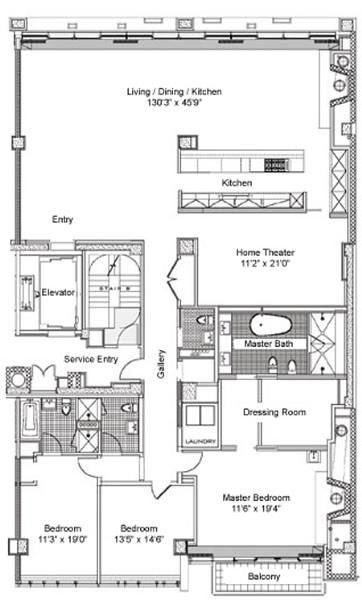This is a detailed blueprint of a residential home, showcasing a meticulous layout. In the bottom left corner, the plan begins with two bedrooms. Adjacent to these rooms, on the right, lies the master bedroom which features an attached balcony. Directly above the master bedroom is a spacious dressing room that seamlessly transitions into the master bath.

Moving slightly to the left from the dressing room, the blueprint denotes a 'gallery', which appears to function as a connecting hallway between various rooms. Adjacent to the gallery is a service entry area, and notably, the design includes an elevator to enhance accessibility.

Beyond the gallery space lies a substantial living area, which integrates the dining and kitchen spaces. The kitchen is marked prominently, suggesting a large and central culinary hub. Below this area, the blueprint reveals a well-designed home theater, providing a space for entertainment.

Every room in the blueprint is meticulously labeled with precise measurements, detailing the exact square footage and ensuring clarity in the overall design. The blueprint itself is rendered in shades of white, gray, and black, with a predominantly white background that accentuates the detailed lines and measurements of the home's layout.